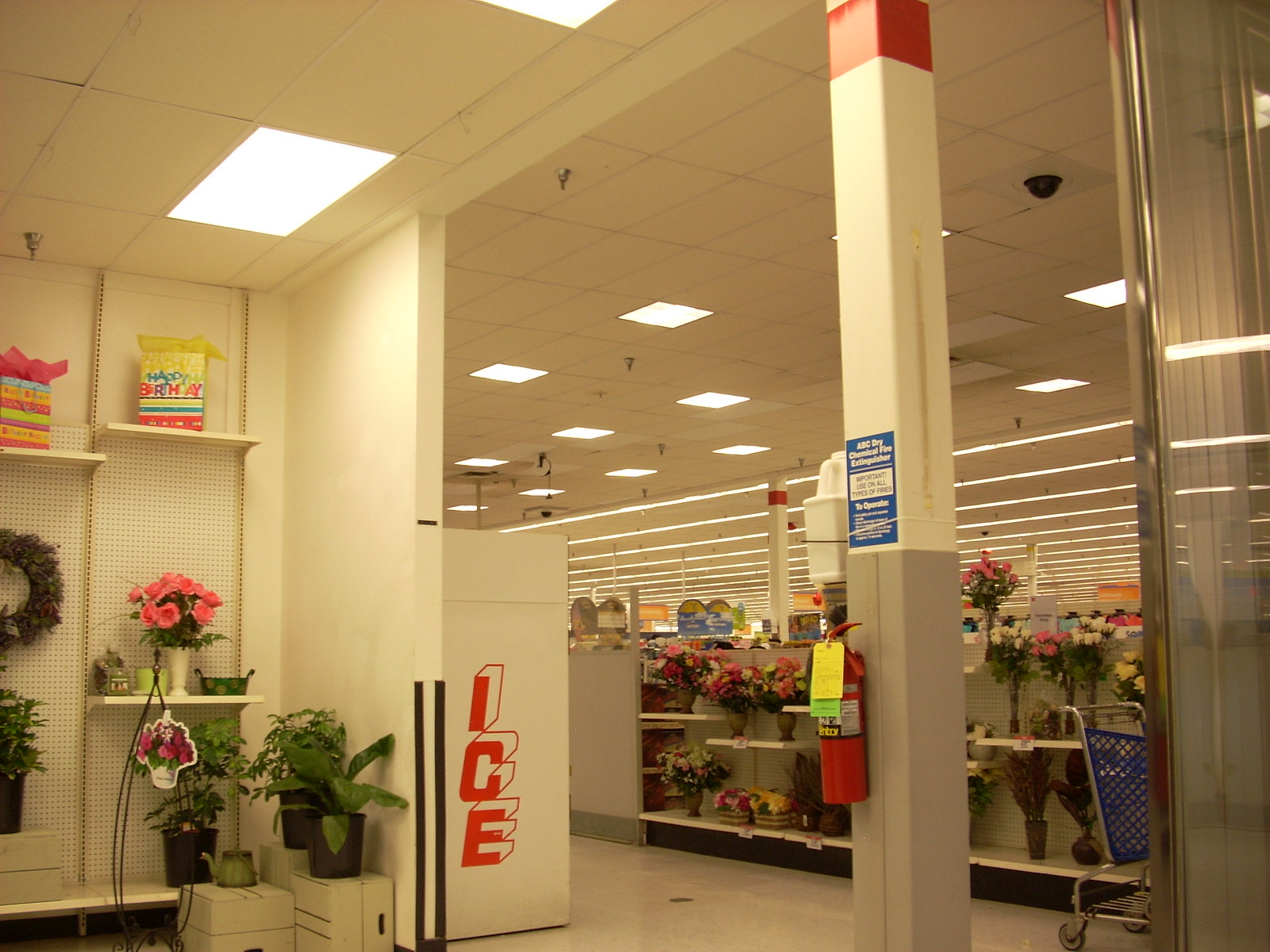This photo captures an indoor sales floor scene in vivid detail. The ceiling features beige-colored ceiling panels interspersed with white fluorescent lights, along with strategically placed sprinklers and a black security camera mounted on one of the panels. The floor is a glossy, reflective white surface. The scene is framed by a doorway or archway with pristine white walls and a white and gray pillar accented with a red strip at the top. Attached to this pillar is a fire extinguisher and a blue and white sign with text too small to discern. To the left of the archway, a vending machine is partially visible next to the wall. Beyond this, white store shelves are lined with various plants in vases, suggesting a mix of artificial and real greenery. In the foreground to the immediate left, the wall hosts a couple of shelves adorned with more potted plants. A blue shopping cart partially enters the frame from the right. The distant view reveals additional ceiling rows of white fluorescent strip lights, illuminating the entire space in a bright, even glow.